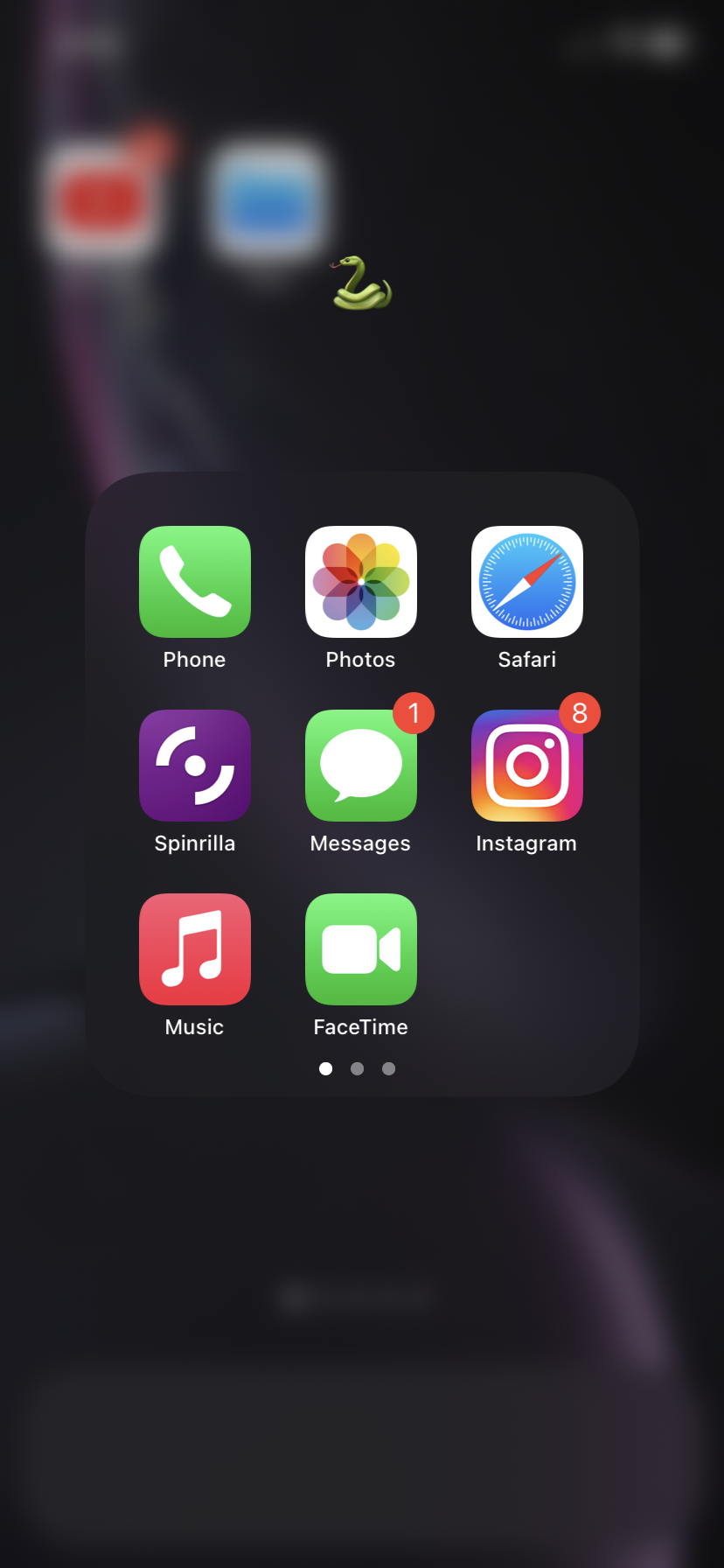This photograph captures the screen of an Apple device, potentially a smartphone or tablet. The background is dark, and at the top, slightly out of focus, is the battery level indicator, hinting that this is a mobile device interface. In the upper-left corner, there are indistinct, blurred buttons, making it hard to identify the exact type of Apple product on display. 

The central portion of the screen showcases a series of distinctly visible app icons, confirming the device's Apple lineage. These icons include Phone, Photos, Safari, Messages, Instagram, Music, and FaceTime, among others. A multicolored flower icon represents the Photos app, and the presence of the Safari browser app solidifies this as an Apple product. Noteworthy details include eight unread Instagram notifications and one unread message notification.

A cartoon image of a coiled snake is positioned at the top center of the screen, adding a unique, personalized touch. At the bottom, a three-dot indicator is visible, with one dot lit, suggesting multiple home screens. While the exact type of device remains uncertain, the visible elements clearly identify it as a member of the Apple family.